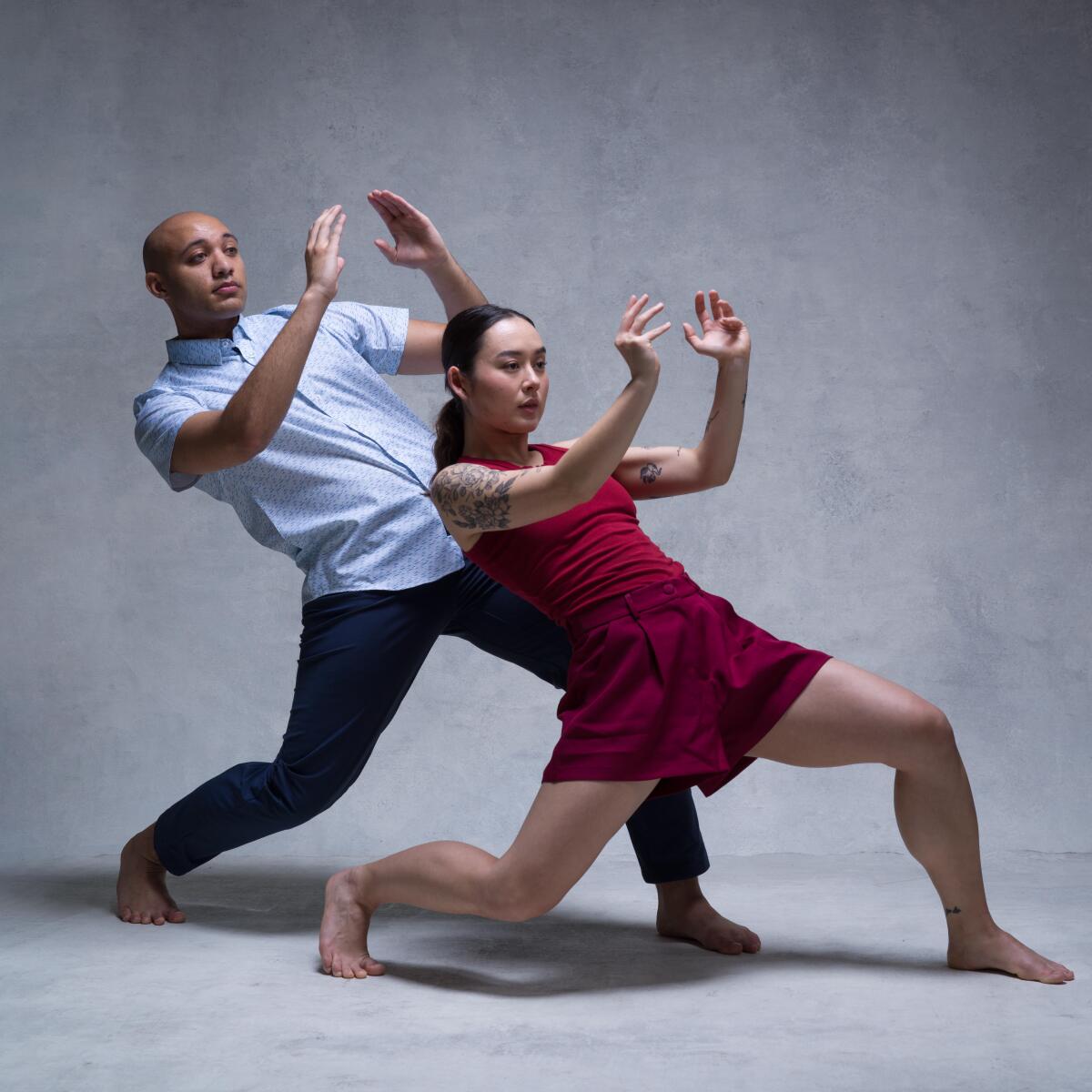In the image, two individuals strike a dynamic pose against a gray studio backdrop with a matching gray floor. Both appear to be of Asian descent and have dark complexions. Positioned behind the woman, the man stands on the left side. He is bald, barefoot, and dressed in a blue short-sleeved button-up shirt along with blue pants. His expression is impassive. The woman, whose full body is visible, stands in front of him, slightly leaned back with her left leg behind her and knee bent. She wears a red tank top and a red skirt buttoned at the waist, revealing tattoos on her right shoulder and left inner arm. Her long black hair is tied back in a ponytail. Both individuals have their hands raised above them as if preparing to hold something, their fingers extended and elbows bent, suggesting a synchronized activity like a martial arts move or a dance routine. Shadow detailing at the top of the image accentuates the studio setting's controlled lighting.